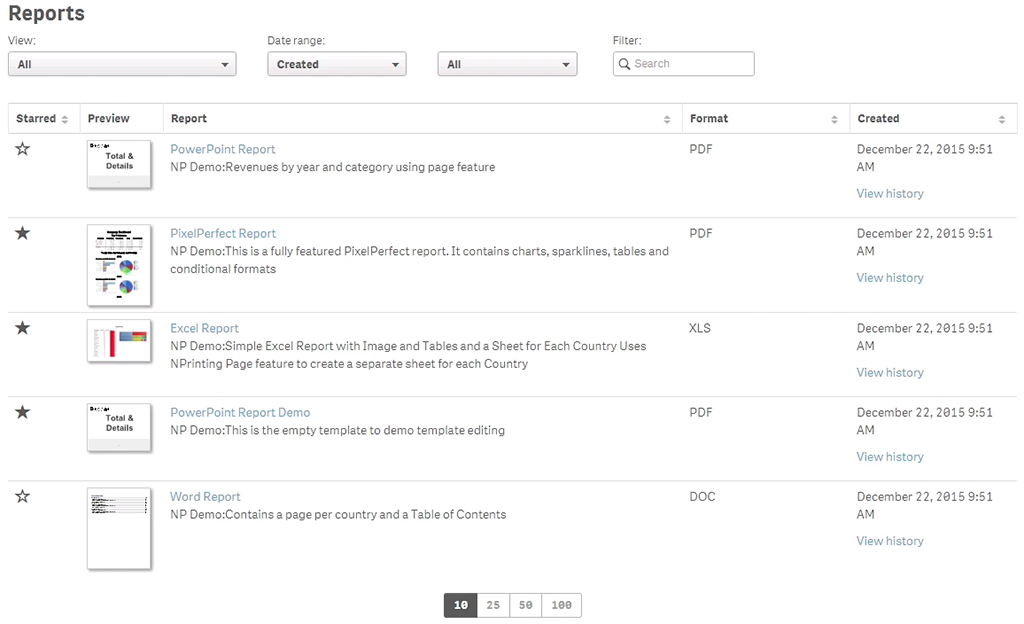The image depicts a user interface of a program focused on generating reports. The interface consists of four drop-down menus aligned in a single row at the top. The first drop-down menu is labeled "View," and it has the option "All" selected. The second menu is labeled "Date Range," and it shows "Created" as the selected option. The third menu simply says "All," with "All" selected, while the fourth element is a filter box where users can input text to refine their search.

Below these menus, the screen is divided into five columns, each representing different report attributes. The columns are labeled "Start," "Preview," "Report," "Format," and "Created," respectively. Each row under these columns corresponds to a specific report.

- In the first column, there is a star icon next to each report title, allowing users to select or deselect the report.
- The "Preview" column contains a small thumbnail image providing a visual representation of the report.
- The "Report" column lists various reports, starting with a "PowerPaint Report" in PDF format.
- The "Format" column indicates the file type, such as PDF, Excel, PowerPoint, or Word.
- The "Created" column provides timestamps for when the reports were generated.

Specifically, the first report is a "PowerPaint Report" in PDF format, created on December 22, 2015, at 9:51 AM. The next report is labeled "Pixel Perfect Report," also in PDF format, created on the same date and time. Additional rows include an Excel Report, a PowerPoint Report Demo, and a Word Report.